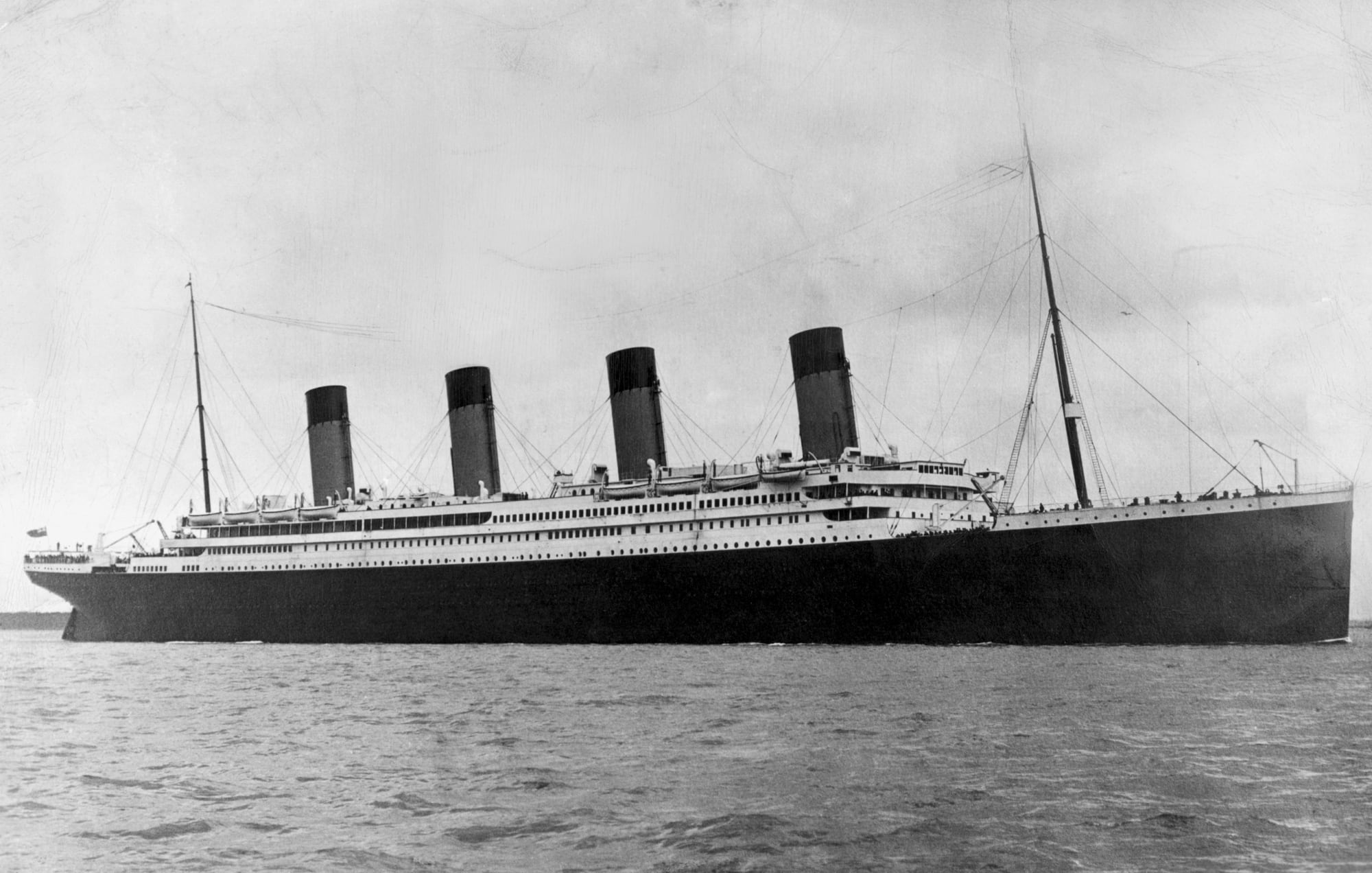This black and white photograph showcases a large, old-fashioned ship reminiscent of the Titanic, situated in the ocean. The vessel, viewed from the side, presents a striking contrast between its dark-colored hull and white upper structure. The ship features two prominent masts—one at the bow and one at the stern—with an intricate network of ropes and ties running along its length. Four substantial chimney stacks rise from the middle of the ship, flanked by lifeboats. At the front and rear of the ship, clusters of tiny figures suggest the presence of people on the deck. The ship's exterior is adorned with numerous windows and portholes, some of which appear to contain glass. A flag, albeit indistinct, is visible at the stern, adding a final touch to this evocative maritime scene.